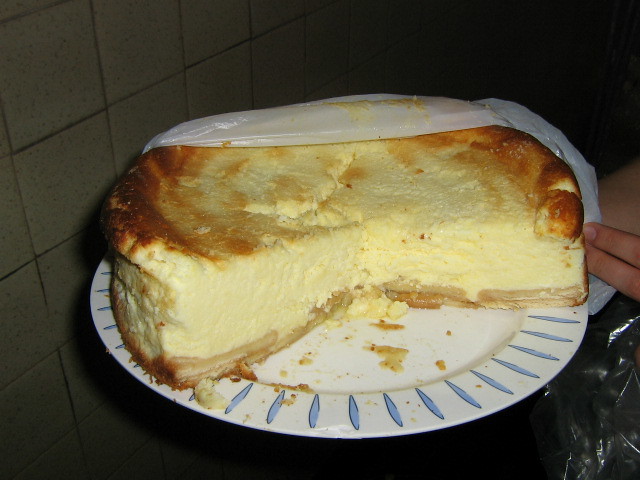The photograph captures an indoor setting, likely a kitchen, indicated by the gray square tiles in the background. Centered in the image is a white plate adorned with blue decorative markings along its rim. The plate is being held by a visible hand, with two fingers prominently pulling back a white piece of plastic wrap that had covered the food item on the plate. 

The focal point of the photograph is a homemade cheesecake, which stands unusually thick at about three to four inches tall. The cheesecake, cylindrical in shape, has a section removed, exposing its creamy, light yellow interior. The top and edges of the cheesecake are a golden to dark brown, indicating it has been well-baked. The area where slices have been taken reveals a scattering of crumbs. The cheesecake looks delectable, suggesting that someone took great pride in presenting and capturing this moment.